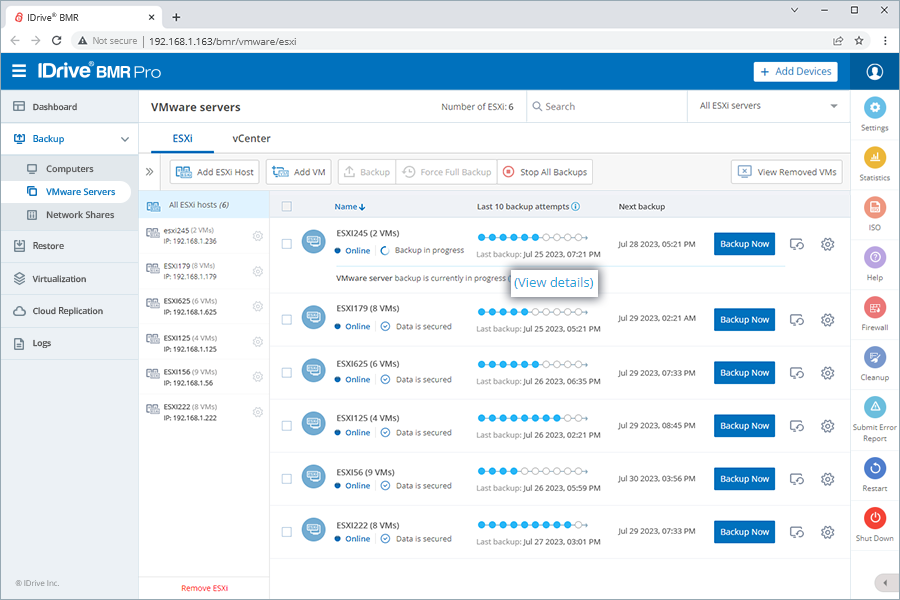An open page of the iDriveVMR Pro interface is displayed, featuring a light gray background complemented by blue headers and buttons, with black and white textual elements. The interface presents a dashboard and various categories such as Backup Computers, VMware Servers, Network Shares, Restore, Virtualization, Cloud Replication, and Logs under the Dashboard section. The current view is focused on the VMware Servers tab, showcasing a detailed window filled with numerous information slots, including data points and dates related to the 'Last 10 Backup Attempts' and the 'Next Backup Attempt.' A prominent blue 'Backup Now' button with white text is available for initiating manual backups despite the automatic schedule. On the right-hand side, a menu provides additional functionalities: Settings, Statistics, ISO, Help, Firewall, Cleanup, Submit Error Report, Restart, and Shutdown buttons.